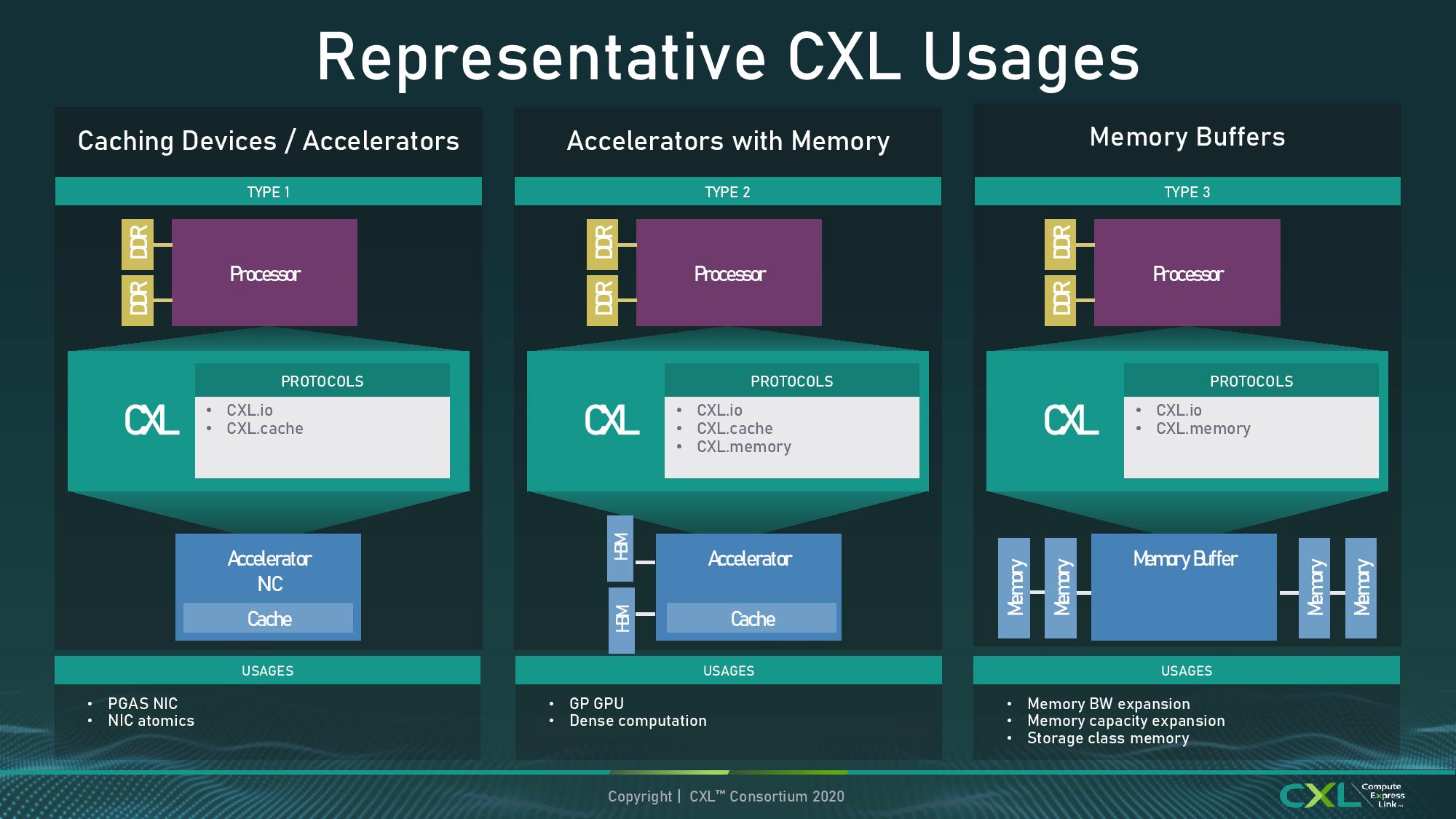The image is a detailed, colorful diagram titled "Representative CXL Usages," showcasing different types of CXL (Compute Express Link) configurations. The layout is divided into three nearly identical columns against a dark green background. Each column, labeled "Type 1," "Type 2," and "Type 3," illustrates distinct computing arrangements: "Caching Devices/Accelerators," "Accelerators with Memory," and "Memory Buffers," respectively. 

Each column starts with a purple rectangle labeled "Processor," from which two yellow rectangles labeled "DDR" extend. Below these, a teal box labeled "CXL" is connected to a white box with a teal header titled "Protocol." The descriptions within these white boxes differ: Type 1 lists "CXL.io, CXL.cache," Type 2 includes "CXL.io, CXL.cache, CXL.memory," and Type 3 mentions "CXL.io, CXL.memory."

At the bottom of each column, a blue box provides further categorization: the first as "Accelerator NC" with a cache beneath it, the second as "Accelerator with Cache" featuring additional blue boxes labeled "HBM," and the third as "Memory Buffer" with blue boxes labeled "Memory." 

Beneath these labels, specific usages are detailed: "PTAs NIC and NIC Atomics" for Type 1, "GP GPU, Dense Computation" for Type 2, and "Memory BW Expansion, Memory Capacity Expansion, Storage Class Memory" for Type 3. The bottom of the diagram includes small gray text stating "© CXL Consortium 2020" and a blue and green CXL Compute Express Link logo on the bottom right.